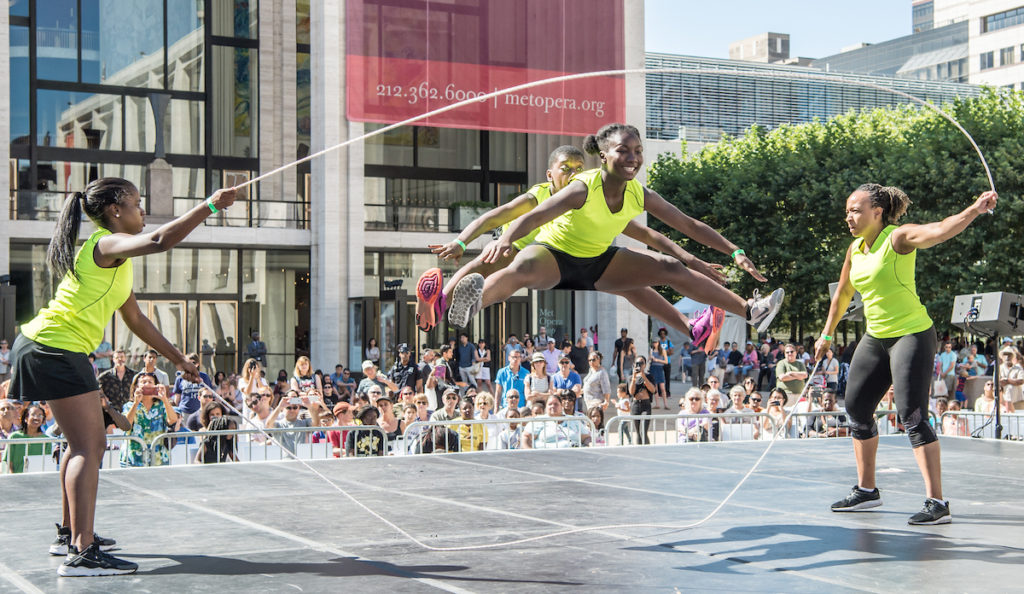The photograph features a vibrant double Dutch jump rope performance by four African-American individuals, comprising three women and one man. The scene is set in what appears to be an urban courtyard, possibly outside a museum or large business complex, with a bustling crowd observing and taking photos in the background. 

The performers are all dressed in matching neon yellow-green tops and black bottoms, though their footwear varies, and the styles of their bottoms include shorts and a skirt. Two women on the outer sides of the image are skillfully swinging the ropes. They both have ponytails and wear coordinated athletic attire, adding to the visual synchrony of the act.

In the center, a man and a woman are energetically jumping in sync, their bodies almost mirror images in their form, with limbs spread out as if in a mid-air split. Their expressions are filled with joy, and they take up the middle third of the photo, drawing the viewer's focus. In the background, a phone number "212-362-6000" and a link to "metopera.org" suggest a possible connection to the Metropolitan Opera or a related cultural event. The entire performance exudes a sense of community, athleticism, and urban vibrancy.